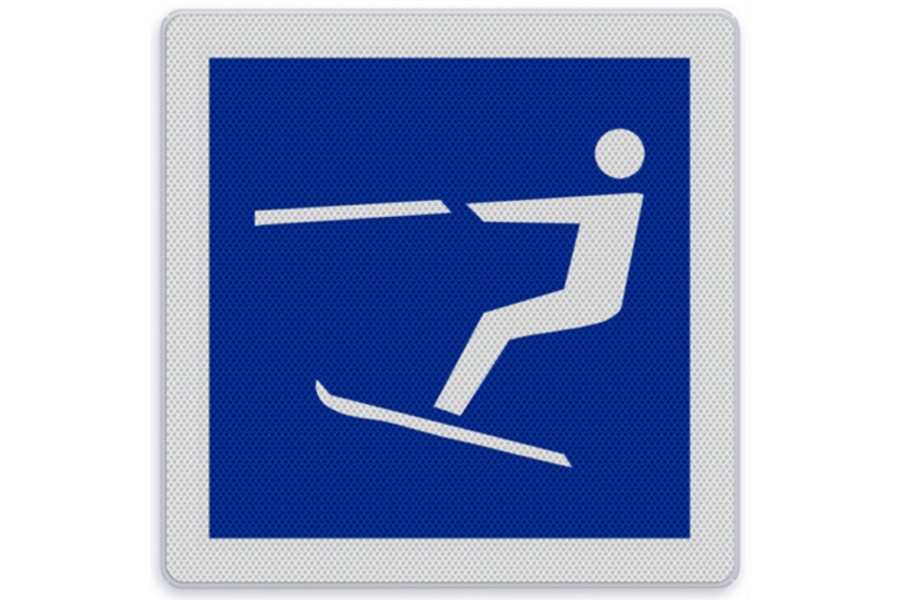The image depicts an icon of a person water skiing against a royal blue background. The figure is simplified into geometric shapes: a circular head and a rectangular body and limbs. The person is facing left, holding onto a horizontal ski pole, suggesting the tension from being pulled by a boat, even though the boat itself is not shown. The person's skis are angled downwards to the right, reinforcing the water skiing action. This graphic is set within a blue square, which is framed by a gray edged border with a white exterior. Both the blue square and the white border appear textured with small, raised dots, adding a tactile element to the visual.